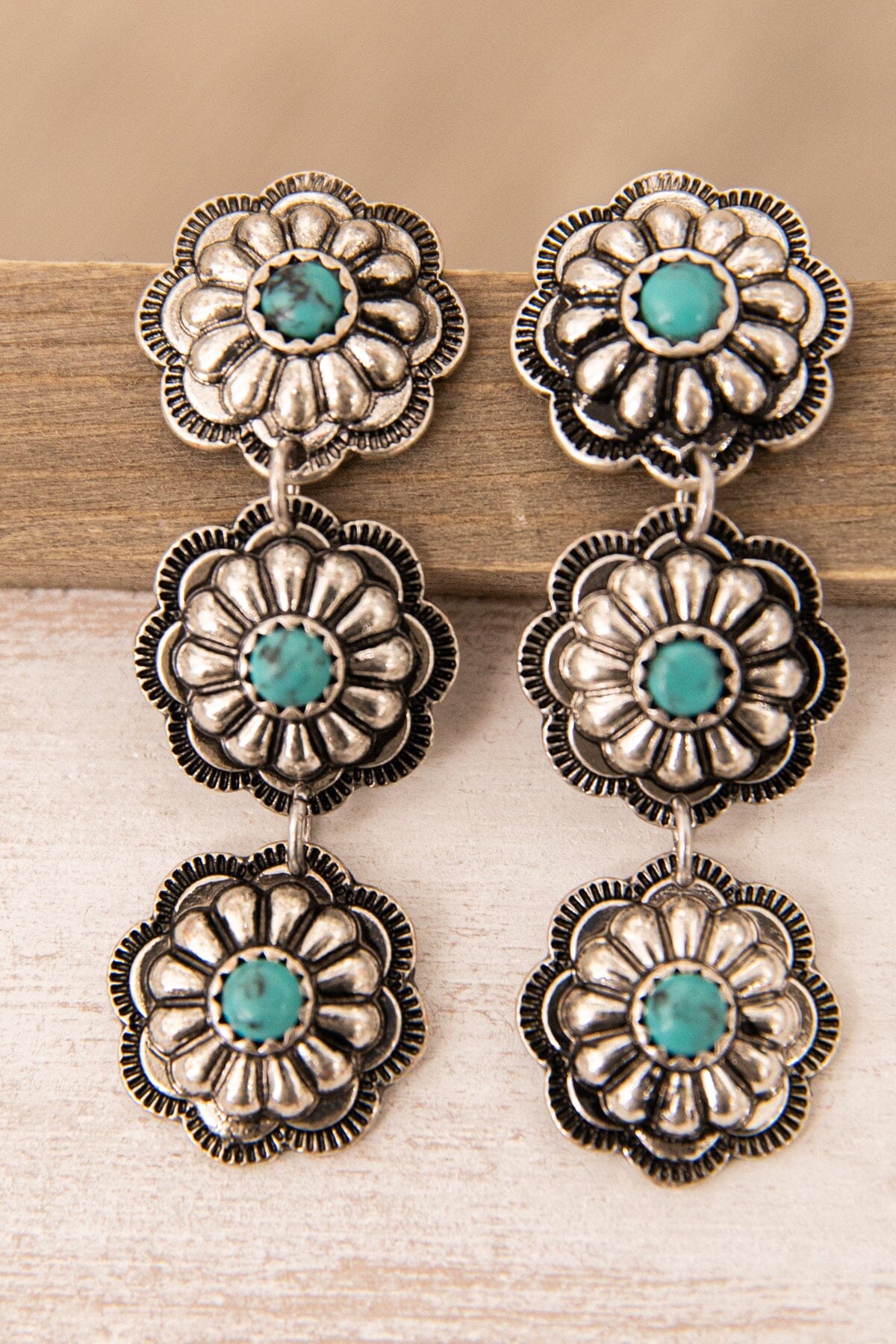This close-up photograph showcases a pair of dangle earrings presented on a vertical rectangular format. The earrings are laid flat against a horizontal wood panel, which occupies two-thirds up the image. Above this panel, the out-of-focus background appears in a brownish-white shade, while below it is an off-white wall. The earrings, identical in design, consist of three vertically linked flower shapes. Each flower features a central round dot of lapis lazuli with a turquoise coloration, surrounded by petal-like structures of all-silver metal. These petals have intricately dimpled black-silver rings outlining them. The earrings are fastened together by silver clasps, creating a harmonious and detailed floral motif with each link showcasing slight variations in the turquoise centers.